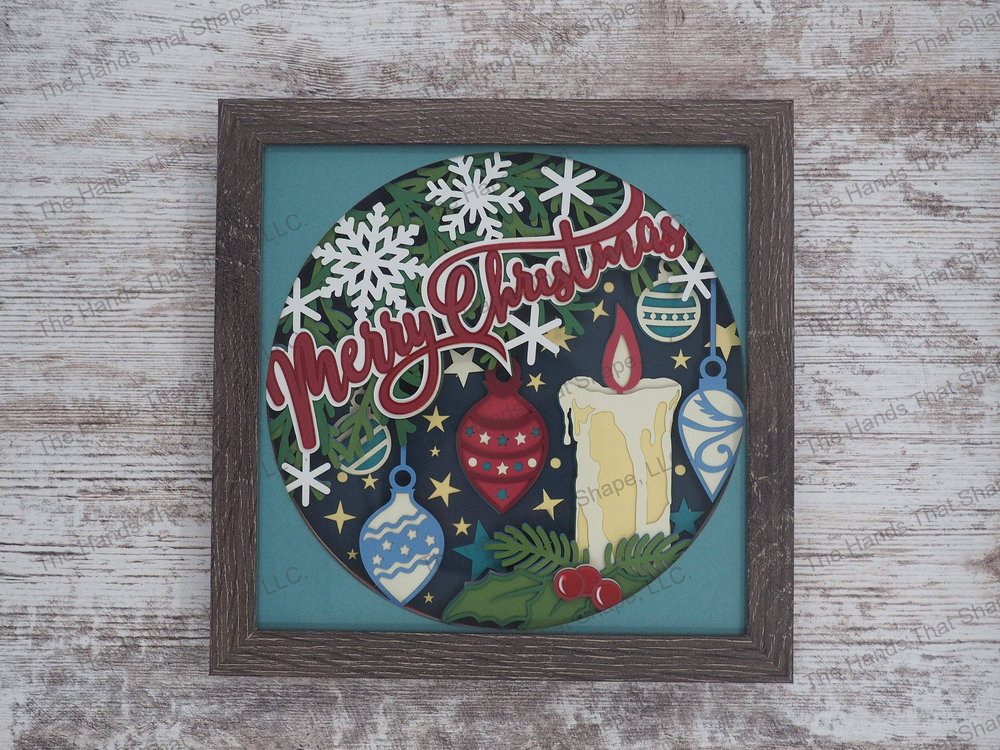This image is a stock photograph featuring a framed artwork with a Christmas motif. The frame, positioned centrally in the image, is made of rustic, dark brown wood and sits on a whitewashed, wooden-style table that is visible on all sides of the frame. Across the image, there is faint, diagonal watermark text that reads "the hands that shape." The artwork within the frame has a light blue background at the corners with a circular design in the center, displaying the words "Merry Christmas" in red cursive. Surrounding the text are various festive elements, including yellow stars, red and blue ornaments, a burning candle with a red flame, holly, green leaves, white flowers, pine tree branches, and large white snowflakes.